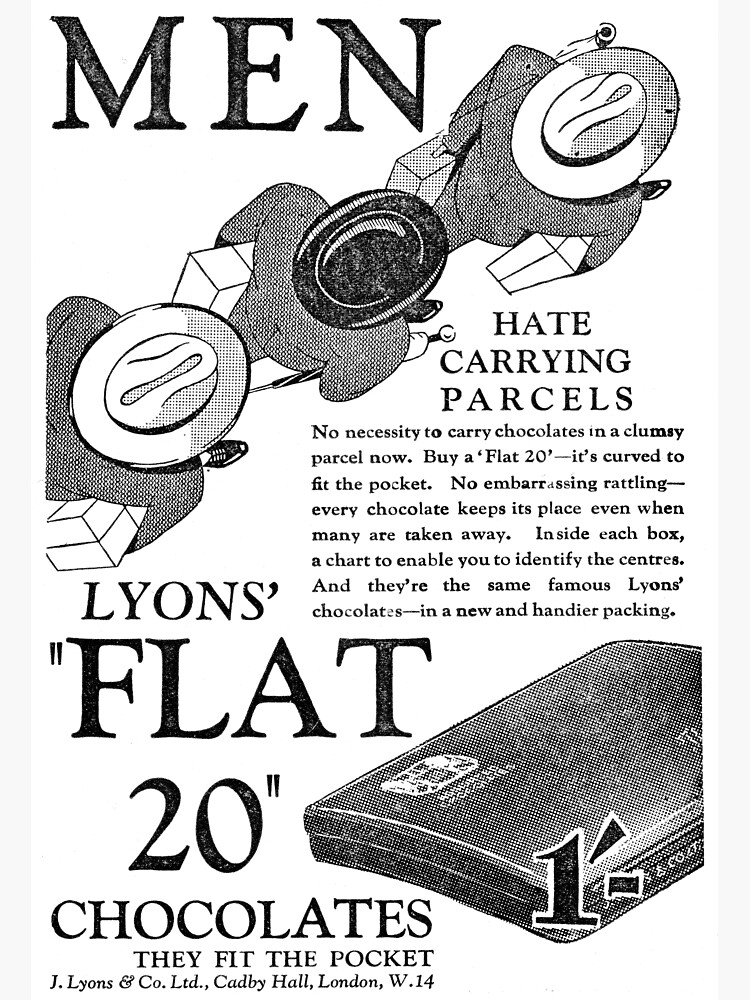This black-and-white advertisement, which appears to be an old magazine page, features a blend of text and illustrations promoting Lion's Flat 20 chocolates. At the top left corner, large black letters spell out "MEN" above a drawing of three men seen from an overhead perspective, each wearing hats and suits reminiscent of the 1920s style. The men are carrying various parcels, likely symbolizing the cumbersome nature of traditional chocolate packaging. Below this image, the text reads, "Hate carrying parcels. No necessity to carry chocolates in a clumsy parcel now. Buy a flat 20, it's curved to fit the pocket. No embarrassing rattling, every chocolate keeps its place even when many are taken away." The advertisement emphasizes the convenience of Lion's Flat 20 chocolates, noting that inside each pocket-sized box is a chart for identifying the chocolate centers. The lower portion of the ad features the manufacturer's details: "Jay Lions & Co. Ltd., Cadbury Hall, London W.14," accompanied by a visual depiction of the chocolate carrying case.